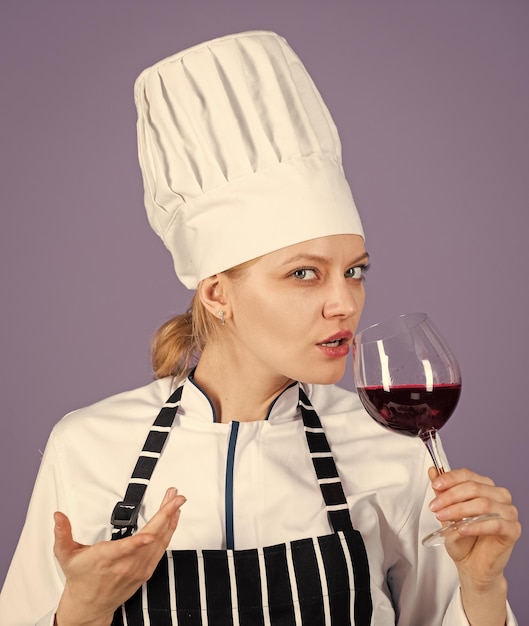This photograph captures a Caucasian woman in her early thirties with fair, almost washed-out skin, blonde hair pulled back into a ponytail, and blue eyes. She wears a pristine white chef's hat and a matching white chef's jacket under a black apron adorned with thin white stripes. Small diamond earrings add a subtle touch of elegance. In her left hand, she holds a half-filled glass of red wine, raising it toward her lips. Her right hand is extended in front of her chest, palm up, as if questioning or expressing something. The backdrop of the scene is a medium to dark lavender hue, lending a soft, muted contrast to the sharpness of her chef's attire. She gazes directly at the camera, blending professionalism with a hint of curiosity in her pose.